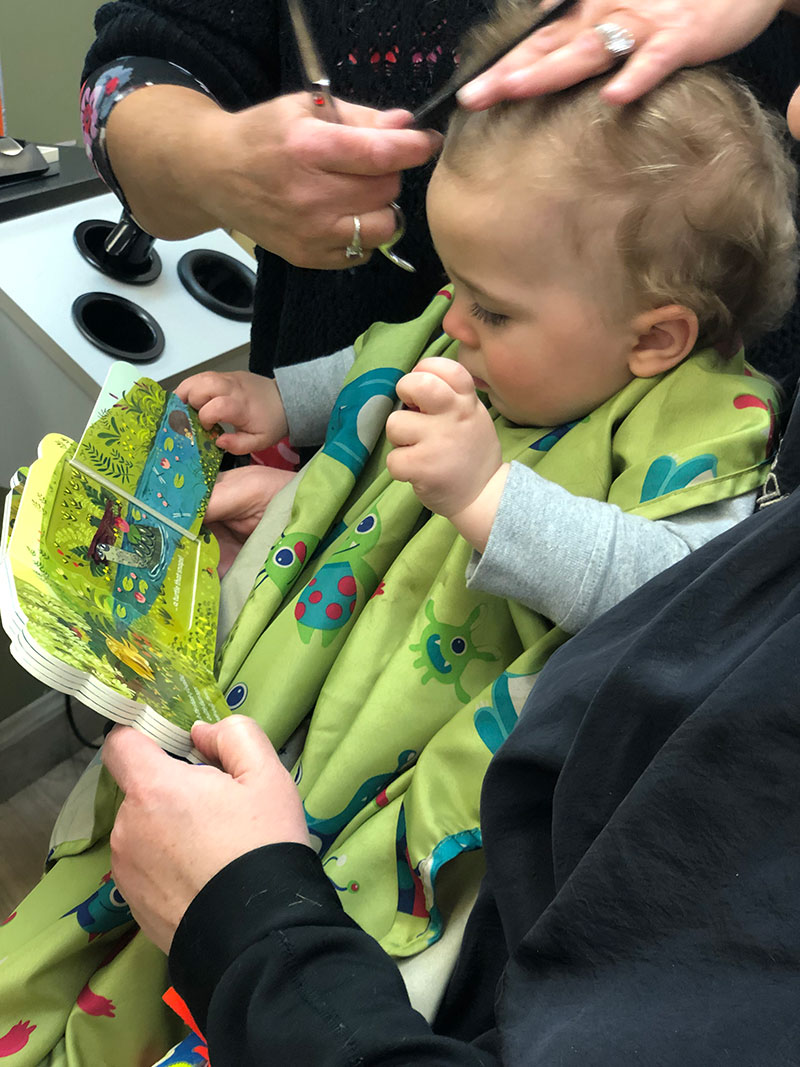The photograph captures a toddler, a white, blonde-haired girl, seemingly around two years old, getting her hair cut. She is clad in a gray sweatshirt with an olive green smock adorned with cartoon characters, which is draped over her and tied behind her neck. An adult, only partly visible with a dark shirt and showing just the chest and hand, is on her right, holding a colorful children's book with thick cardboard pages and fold-out illustrations that the toddler is attentively engaging with, especially a vivid page depicting water creatures like crocodiles and frogs amidst a leafy pond scene. In the background, a white woman hairstylist, dressed in a dark smock and wearing a few rings, is visible, holding a comb and scissors as she delicately works on the toddler's hair. The setting includes a holder with various hair-cutting instruments along the wall behind the hairstylist. The toddler appears engrossed in the storybook, calmly distracted from the haircutting process.